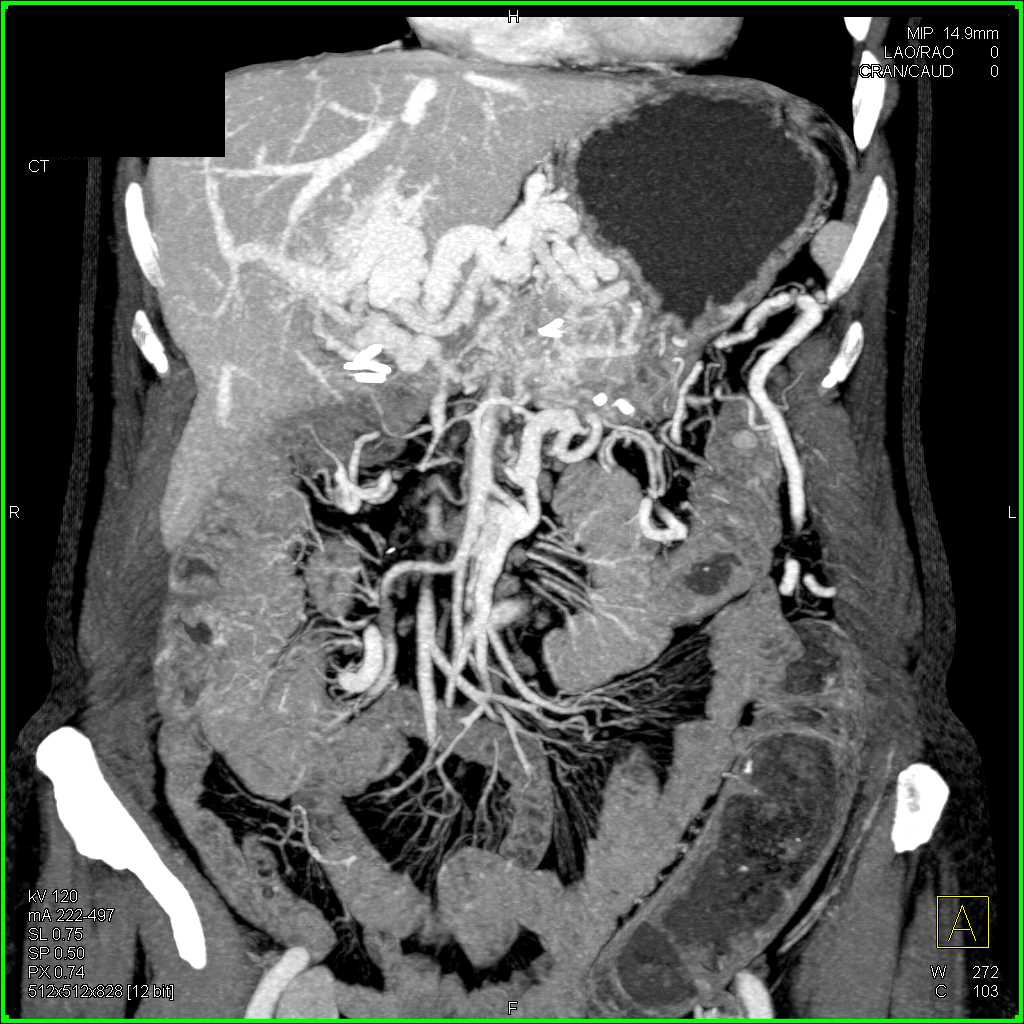This black-and-white photograph, possibly a technical scan or X-ray, shows the complex interior of what appears to be a human body, though it could also be an animal's. The image intricately depicts various internal organs and structures. Dominating the scene are the large and small intestines, surrounded by a network of winding tubes and blood vessels. The tubes vary in size and shape; some are long and tube-like, while others split into finer, hair-like figures. The organs and structures are highlighted in shades ranging from white to charcoal, providing contrast against the darkened background. On the left, the liver is visible in a light gray hue, and layers of muscle and skin can be seen throughout the edges. Additional anatomical details include leg muscles and bones at the periphery. Significant markings, such as "MP14.9N," are noted at the top-right corner, further indicating the technical and diagnostic nature of this scan.